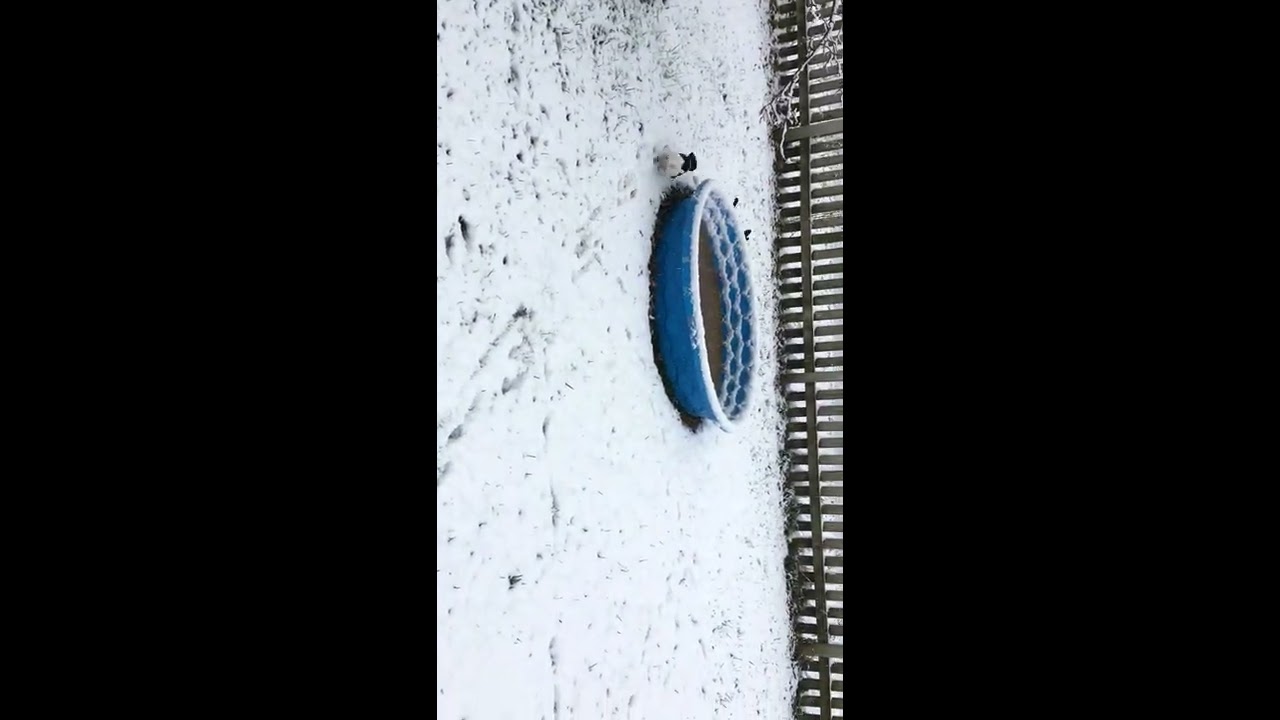This sideways photograph captures a snowy backyard scene in the middle of winter. The ground is blanketed with snow, though patches of grass and a few leaves are still visible. Dominating the center of the image is a small, round kiddie pool, blue and white in color, about two to three feet wide. A thin layer of snow rests on top of the pool, with a bit of water inside it. In the background, a brown slatted fence extends across the length of the photograph, with light filtering through its gaps. The photo, taken during daylight, vividly showcases a serene yet somewhat neglected winter landscape.